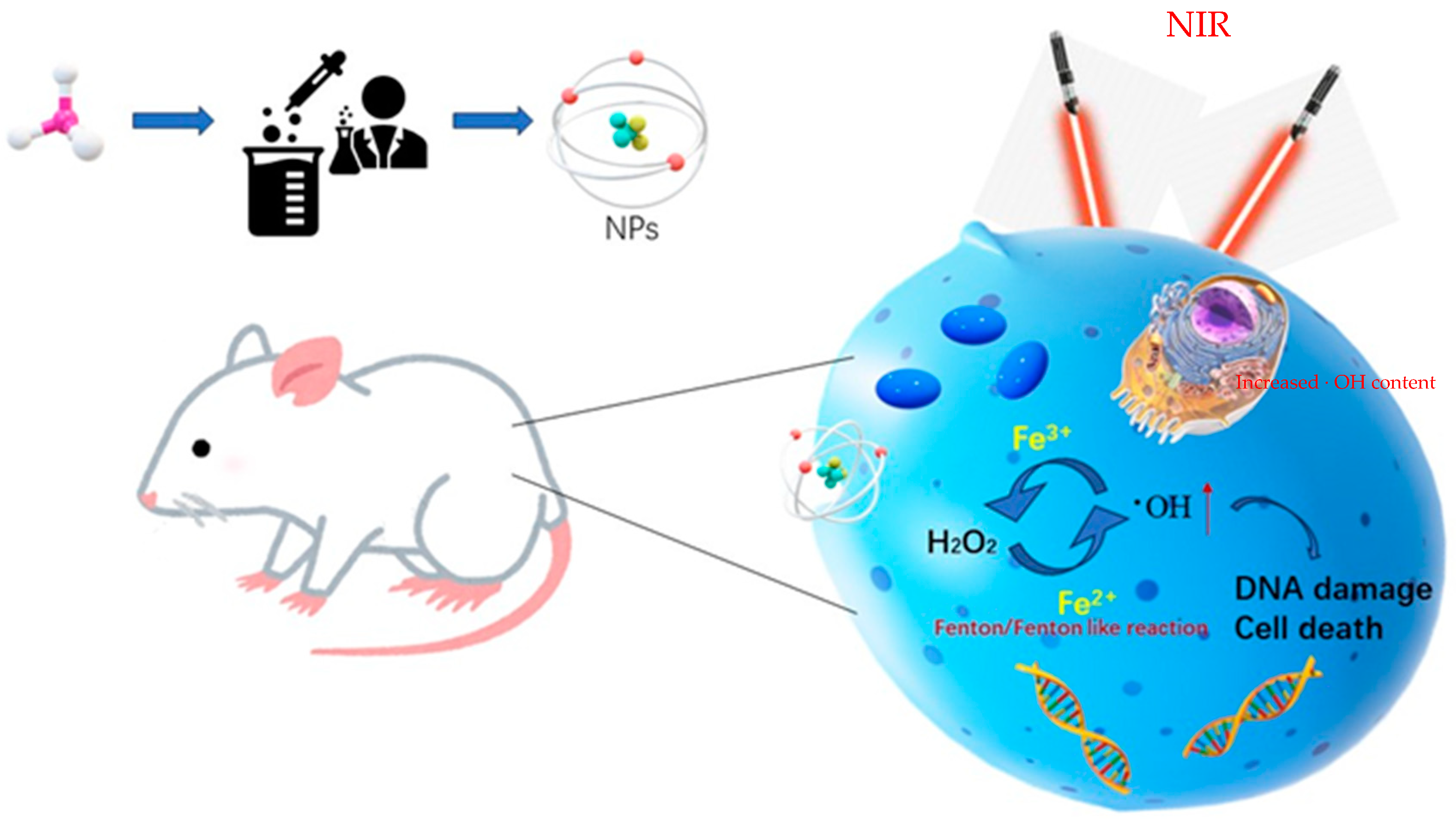This detailed scientific diagram illustrates a sequence of events in a biological experiment involving a mouse and DNA manipulation. At the top, a cell is depicted with a blue arrow pointing to the right, indicating movement towards a beaker with a dropper overhead, which is controlled by a scientist holding another beaker. Following this, another blue arrow leads to a white helix surrounded by colorful dots, labeled with the letters "NPS." Below this, a white mouse with a gray outline, pink feet, tail, and ears is shown. Two lines extend from the mouse to the right, pointing towards a large blue blob containing DNA sequences and cellular structures, labeled with "DNA damage" and "cell death." The blue blob also includes symbols and labels such as H2O2 and OH, indicating chemical components involved in the experiment. This diagram effectively combines visual and textual information to represent the process and outcomes of the experiment.